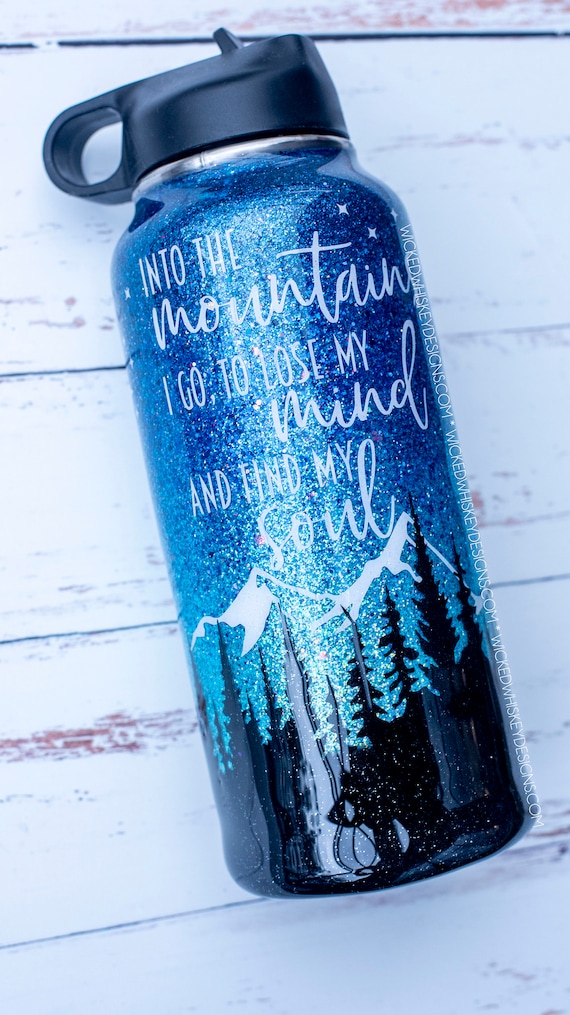A detailed photograph showcases an intricately designed drinking bottle resting on a light-toned wooden surface. The bottle features an inspiring quote in a mix of white cursive and print that reads, "Into the mountains I go to lose my mind and find my soul." The background of the bottle displays a mesmerizing gradient, transitioning from a predominantly sparkly blue to a blend of teal and aqua. Snow-covered mountains in blue hues dominate the middle section of the design, adding a touch of serene nature. In the foreground, silhouettes of dark trees create a striking contrast. Scattered white stars adorn the backdrop, adding a celestial touch. The bottle is topped with a black lid that includes a practical circular handle, perfect for attaching to a backpack. It also features a pull-up straw and a tiny strip of silver just beneath the black lid, hinting at its functionality and style.